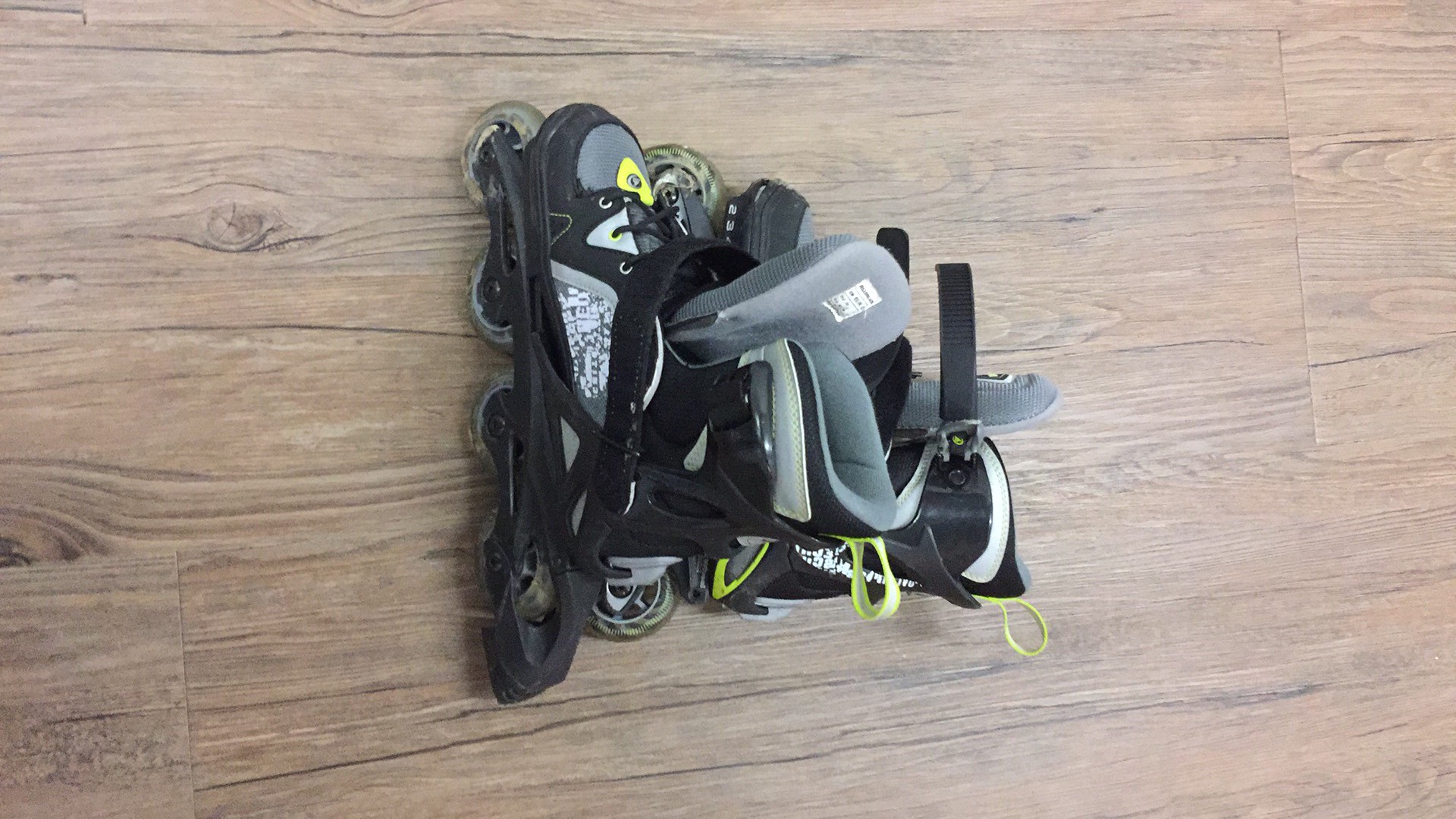This is an overhead photo of a pair of black and gray rollerblades placed on a wooden floor with dark brown accents. The rollerblades each feature four wheels aligned in a straight line, with the wheels appearing somewhat dirty and transparent. The skates are standing upright, with the toe parts facing the upper section of the image. Notable details include fluoro yellow loops on the back of each boot, designed to help pull the skates onto the feet. The skates incorporate black plastic bottoms, black laces, and gray foam tongues and interiors. Additionally, there is a large piece of plastic extending from the back of each skate, which serves as a brake.